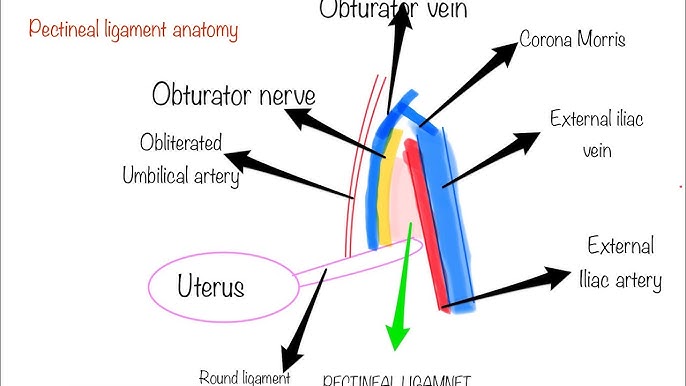The image is a detailed and simplified anatomical drawing titled "Pectineal Ligament Anatomy," focusing on the uterus and surrounding structures. The uterus is highlighted with a pink outline, while various other parts are marked with different colors such as blue, red, and yellow. Key components indicated include the obturator nerve, obliterated umbilical artery, obturator vein, corona moris, external iliac vein, and external iliac artery. Black arrows point to these elements, creating a clear guide through the anatomy depicted. The drawing primarily uses splashes of color to denote the relative locations of these structures, with text labels for each.